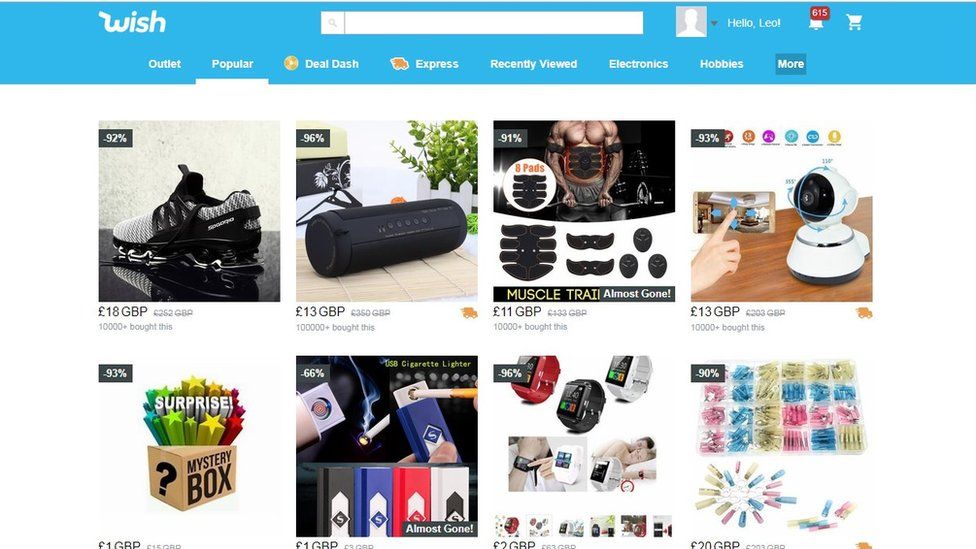The website displayed is Wish.com. At the top, there is a light blue header with the "Wish" logo in white. Next to it, there's a search bar and an account icon, showing "Hello Leo." A red notification bubble with the number 615 is visible above the bell icon, indicating notifications. The shopping cart icon is empty.

Below the header, there are several tabs: "Outlet," "Popular," "Deal Dash," "Express," "Recently Viewed," and more. The "Popular" tab is currently selected.

The webpage features various items:
- A shoe priced at £18.
- A speaker priced at £13.
- A muscle toner device, priced at £11, which appears to be almost sold out. This device can be strapped to the stomach and connected to weights via a barbell.
- A small fan or possibly a pan for £13.
- A surprise box for £1.
- A cigarette lighter for £1.
- An unidentified item, possibly a wrist alarm.

Each item displays its price and some have a limited time offer indicated. The visual layout prominently features the items with clear images and prices in pounds, reflecting a UK-based interface.